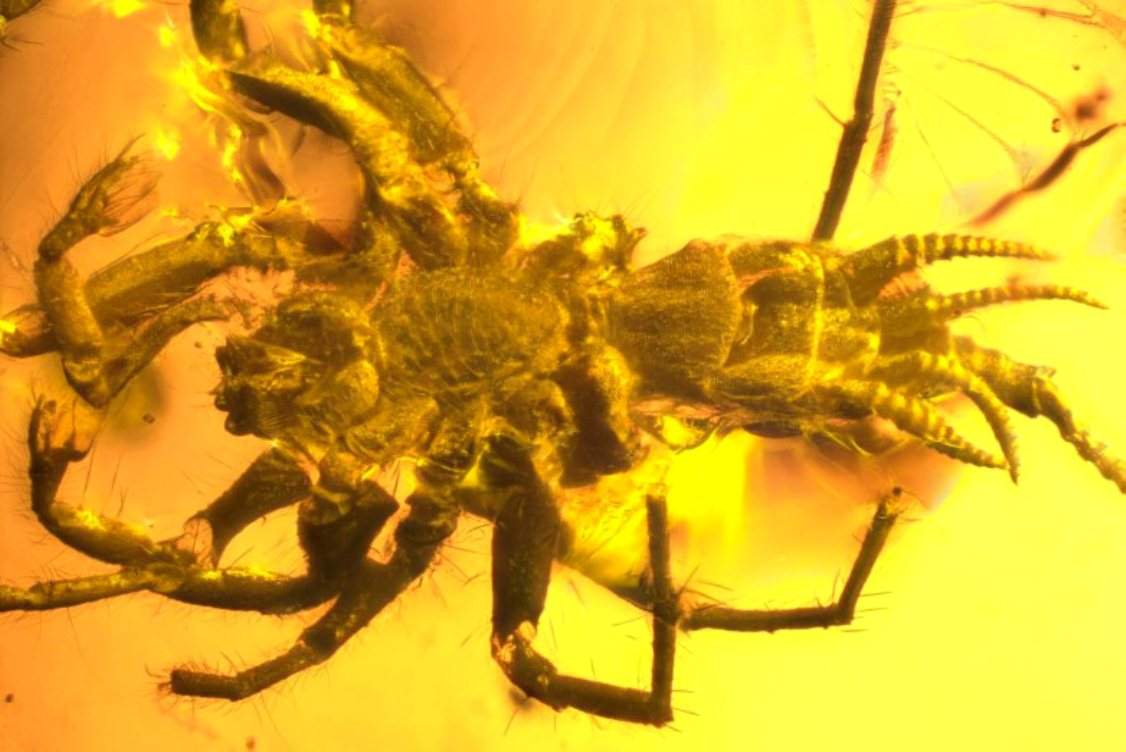The image depicts an up-close view of an arthropod, possibly a shrimp, lobster, or crayfish, photographed from below. This creature takes up most of the frame, displayed against a vivid background that transitions from bright neon yellow at the rear to a darker orange hue towards the head. The animal's lower body appears to be disintegrating, whereas the upper part features eight spider-like legs and blurred hairs protruding from its appendages. The thorax culminates in a distinctive growth with appendages resembling claws or tails. Its eyes are visible on the head, which somewhat resembles the top of a frog's head. The entire scene is slightly out of focus, emphasizing the creature's decaying state and creating a dramatic contrast with the brightly lit tank background, possibly indicating it's in a tank designed for selection, perhaps for culinary purposes.